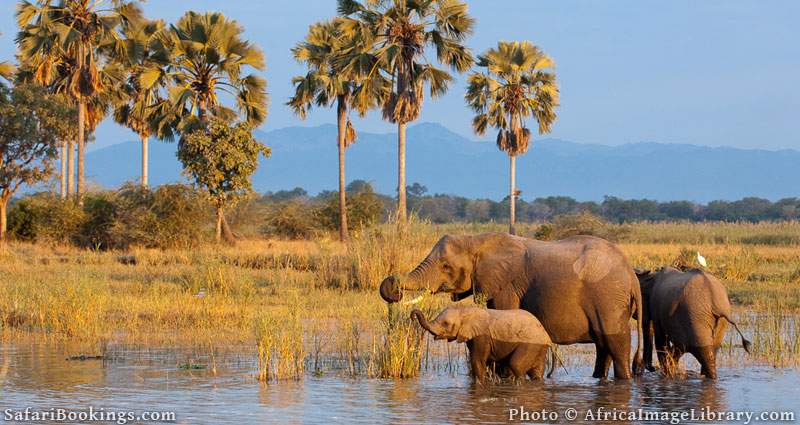In this vibrant outdoor photograph, we see a serene natural setting featuring a field lush with green and yellowish grass interspersed with water pools. Centered in the image are three brown elephants, partially submerged as the water reaches only as high as their legs. Among the trio, two are adults—a probable mother and another larger elephant—while a smaller, young calf stands close by. Notably, a small bird, likely a seagull, is perched atop the back of the third elephant. The elephants appear to be drinking or possibly grazing on the abundant vegetation within the water. Surrounding this tranquil scene, the backdrop reveals an array of tall palm and coconut trees, and far off, the hazy silhouette of a mountain range accentuates the scene's depth. Above, the sky is a clear blue, adding to the picturesque quality of the landscape. In the bottom corners of the image, text indicates it is sourced from SafariBookings.com and copyrighted by Africa Image Library.